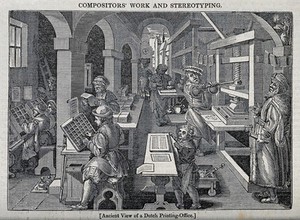In this black and white drawing that suggests an old-time setting, we observe an intricate indoor scene depicting a bustling factory workshop. The detailed artwork reveals numerous figures actively engaged in various tasks, ranging from operating mechanical machines to writing and monitoring activities. Notably, the crowd includes smaller individuals, possibly resembling leprechauns, contributing to the industrious atmosphere. The room, adorned with arches and a window providing natural light, appears well-maintained and more aesthetic rather than purely utilitarian. The image is framed by a grey border, with the title "Compositor's Work and Stenotyping" prominently inscribed at the top center, although the text at the bottom center remains too faint to decipher.